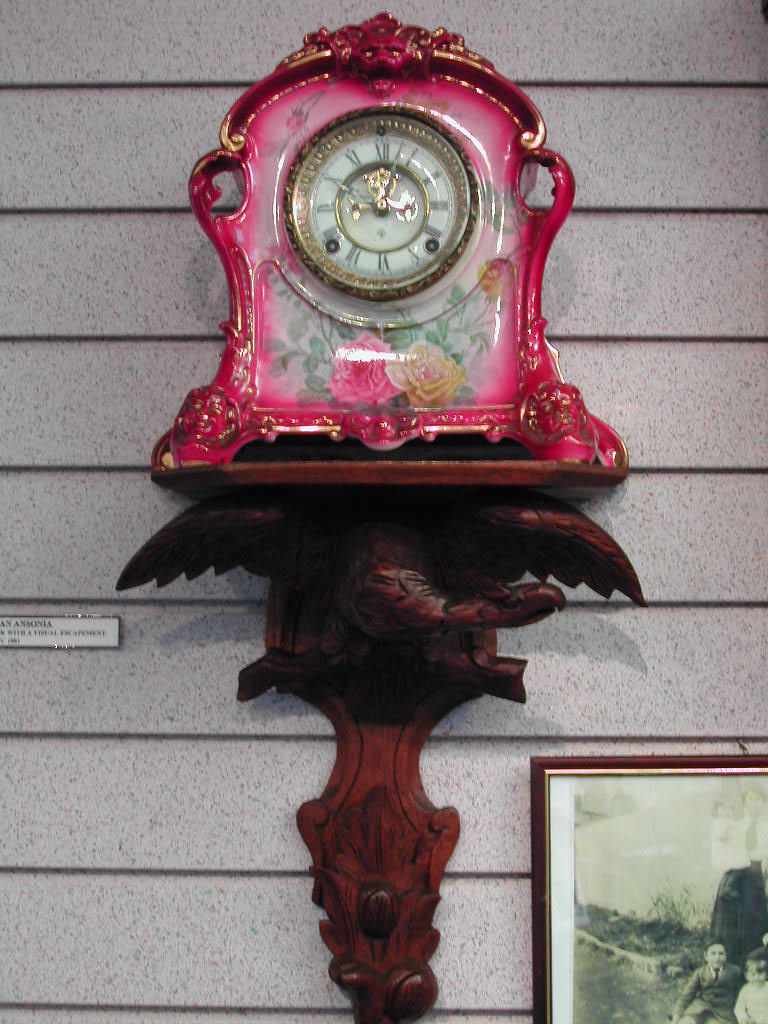This image features a beautifully detailed Miami cuckoo clock mounted on an intricately carved wooden shelving unit. The clock, notable for its antique charm, stands out with its Roman numerals (I through XII) encircling the clock face. The timepiece is adorned with a distinctive pink and white color scheme, embellished with delicate floral patterns. Topping the clock is a unique gargoyle ornament, adding to its eclectic design. Positioned next to a painting, the clock is accompanied by a small plaque with an inscription, further hinting at its historical or sentimental value. The setting, possibly a store, includes a textured wall which complements the overall vintage aesthetic of the display.